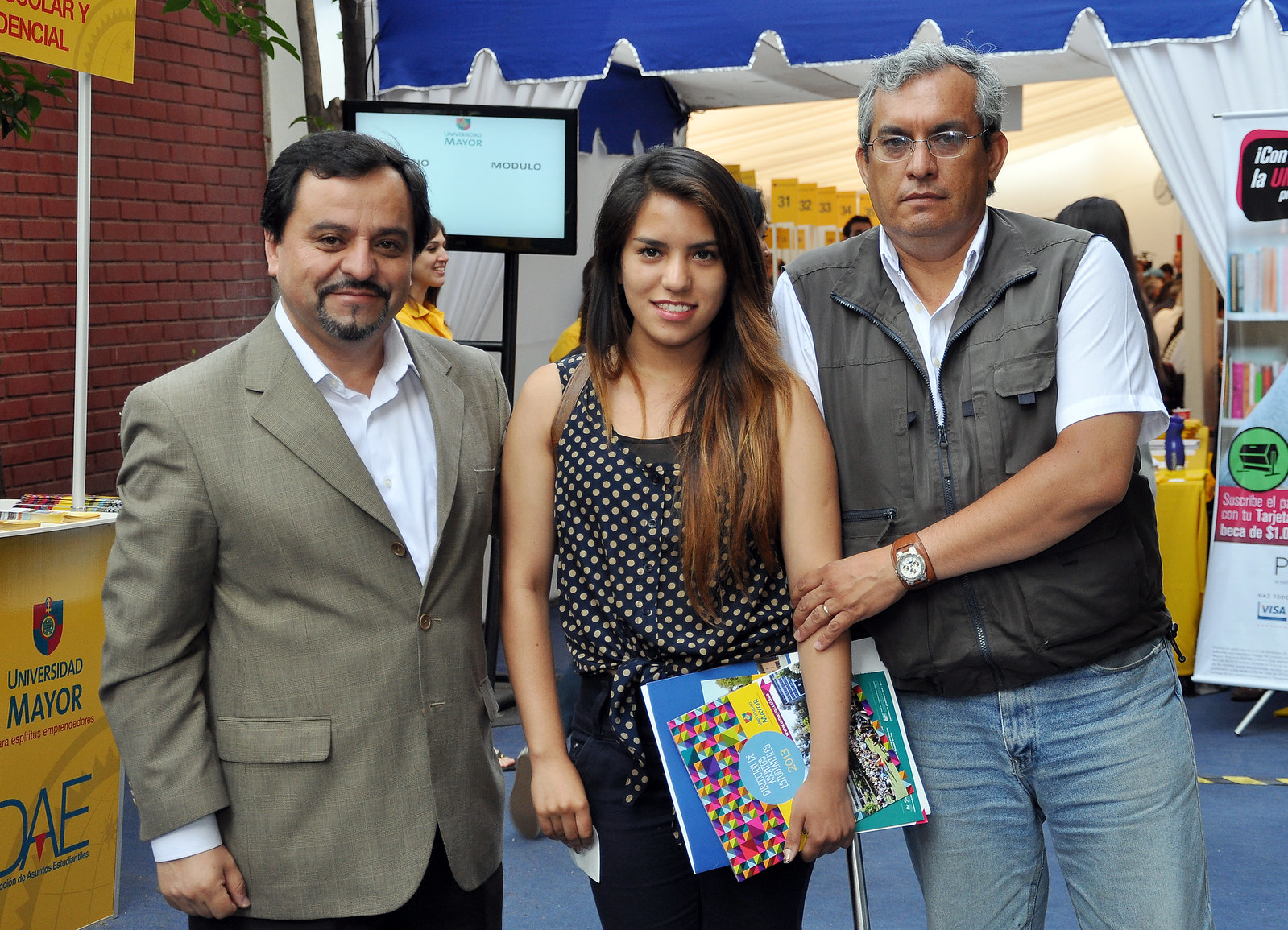In this outdoor photograph, three individuals are captured prominently against a backdrop suggestive of an expo event. On the right stands an older gentleman with glasses, dressed in a white shirt, a gray vest, and blue jeans. He exudes a casual yet refined style. At the center is a young woman with brown hair transitioning to a lighter shade at the ends. She is attired in black pants and a black shirt adorned with small decorative elements, holding a book and a pamphlet, perhaps gathered from the event. To her left is a middle-aged man sporting a gray suit jacket over a white shirt, paired with charcoal-colored pants. He has a distinguishing mustache and a small beard, complemented by his dark hair. The background features a booth and a brick wall with a stand, indicating a setting aligned with an exhibition or a similar gathering.